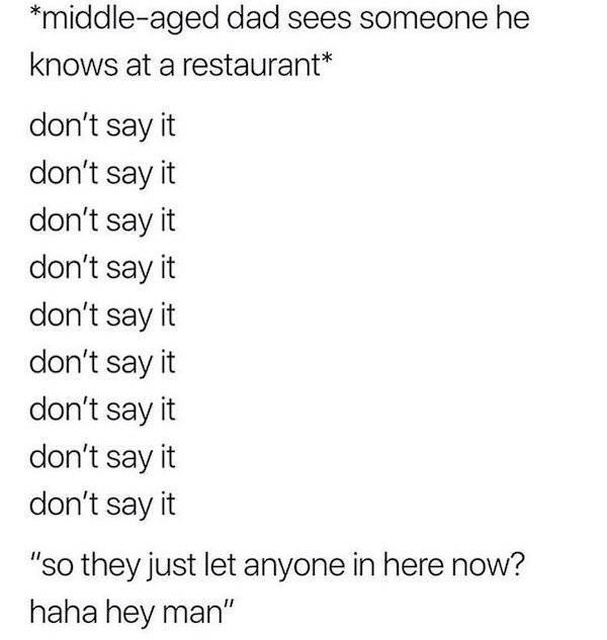This meme features a minimalist design with a simple white background and black text. The content is formatted as follows:

- On separate lines, an asterisk is followed by the text: "*Middle-aged dad sees someone he knows at a restaurant.*"
- After a brief pause indicated by a scroller symbol, the meme continues with repeated lines, each separated by a page break: "Don't say it. Page break. Don't say it. Page break. Don't say it. Page break. Don't say it. Page break. Don't say it. Don't say it. Page break. Don't say it. Don't say it. Page break. Don't say it."
- Finally, the meme culminates in a classic dad joke, presented within quotation marks: "They just let anyone in here now. Haha, hey man."
  
This humorous text-only meme relies on the familiarity of dad jokes and the predictable nature of dad humor to elicit a chuckle. The entire meme is devoid of images, doodles, or graphics, emphasizing the simplicity and effectiveness of text-based humor.